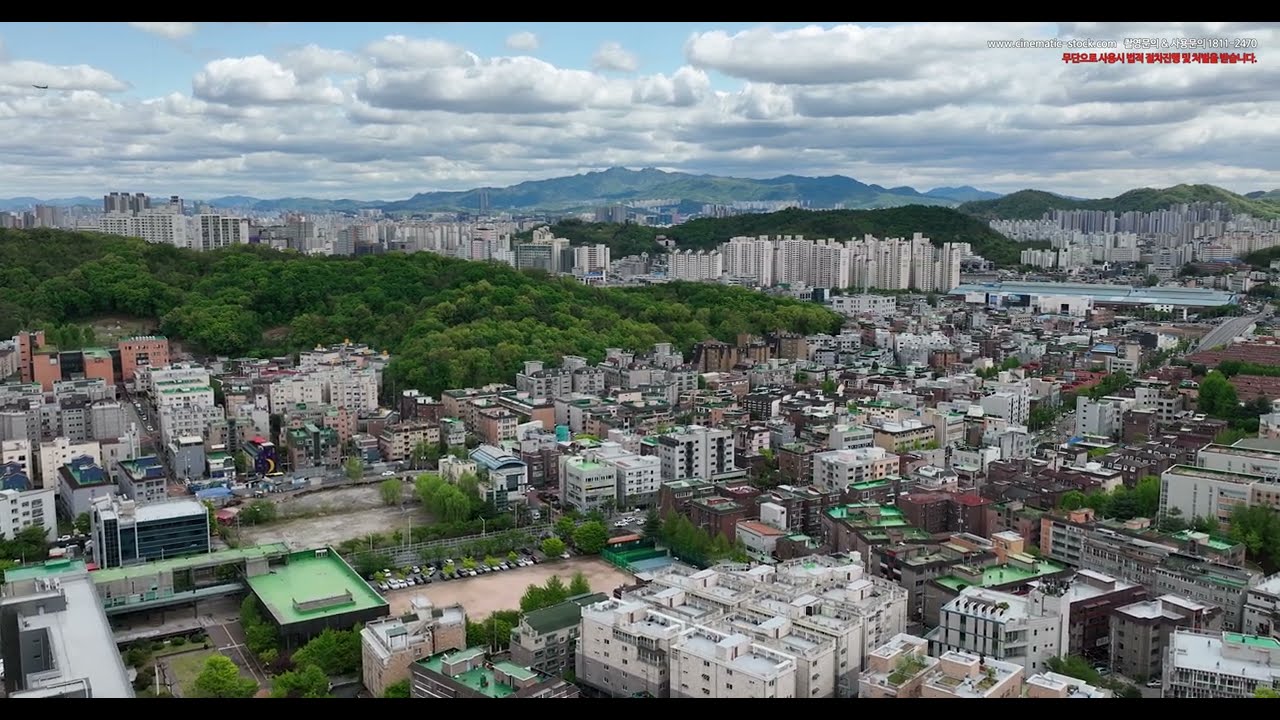An aerial photograph captures a sprawling, vibrant city situated amid rolling hills and a mountain range in the background, under a partially cloudy blue sky. The city showcases a diverse architecture predominantly featuring white buildings, with a mixture of other colors adding to its charm. Tall buildings populate the background, but they're not quite skyscrapers by global standards. The foreground displays a more traditional cityscape with smaller, multi-story structures interspersed with greenery and trees. A river runs through the right side of the image, flanked by high-rise buildings. The top right corner of the image is marked by a URL, "www.cinematicsstock.com," and additional white and red text in an Asian script, suggesting the city might be located in Asia. The stunning realism of the drone-captured image highlights both the city's expansive nature and its intricate details.